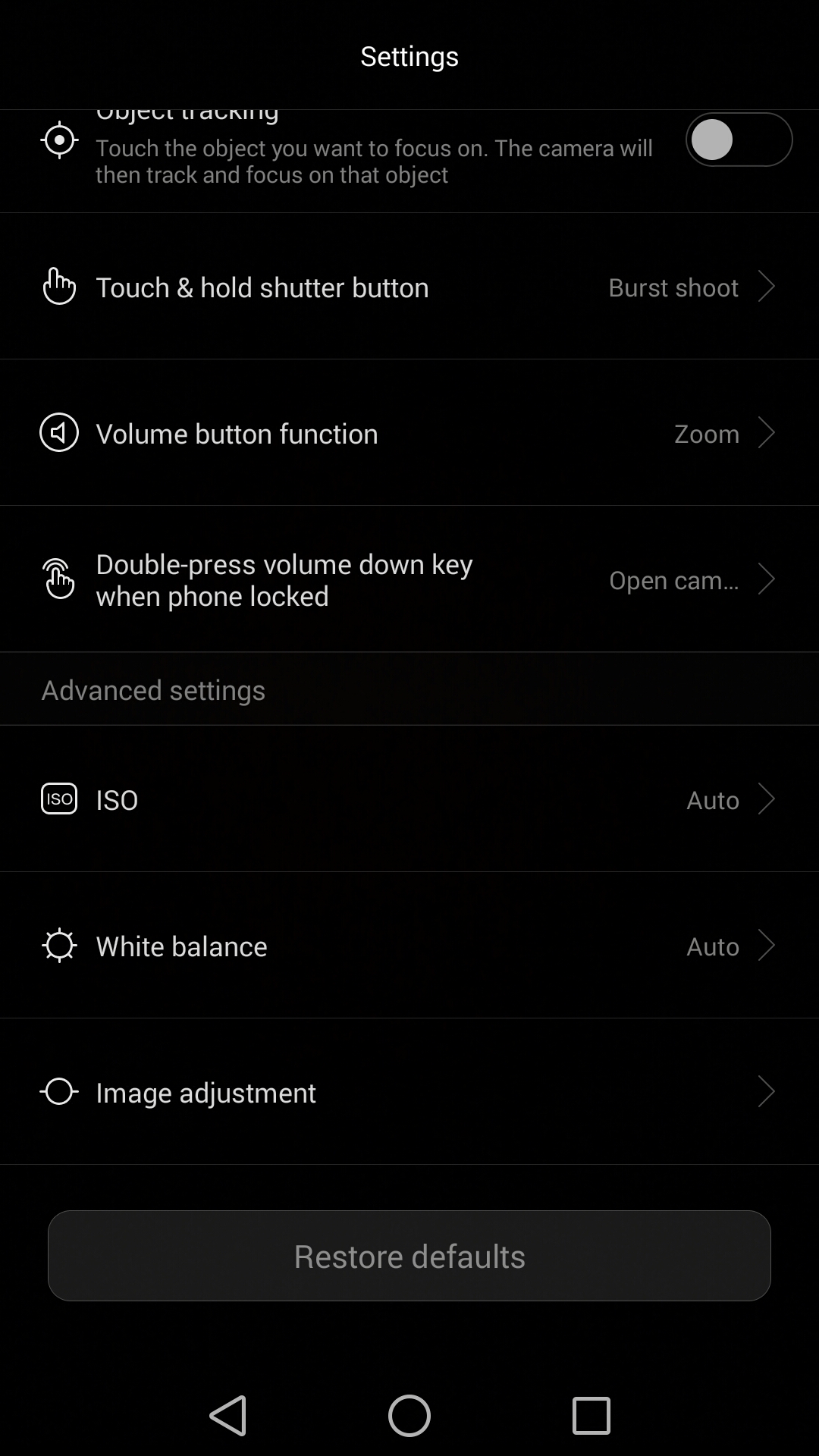This image appears to be a screenshot from a smartphone's camera settings menu. The background is black, adorned with white text to clearly delineate various categories and options. In the settings menu, you first encounter partially visible instructions due to some text being cut off, which seem to direct the user to "touch the object you want to focus on," allowing the camera to track and focus on that object. An additional note explains that this feature isn't currently activated.

Further options include:
- **Touch and Hold Shutter Button**: Enables burst shooting mode when held.
- **Volume Button Function**: Set to zoom.
- **Double-Press Volume Down Key When Phone is Locked**: Set to open the camera.

The "Advanced Settings" section features parameters such as:
- **ISO**: Automatically adjusted.
- **White Balance**: Also set to auto.

There is an option for "Image Adjustment" marked by a right arrow, suggesting that additional settings can be accessed through this menu.

At the bottom of the interface, there's a gray box labeled "Restore Defaults" for resetting settings to their original state. Standard navigation icons populate the very bottom section of the screen, providing ease of access to other features of the phone. The use of contrasting colors - white text on a black background with gray elements for emphasis - ensures readability and user-friendliness throughout the menu.